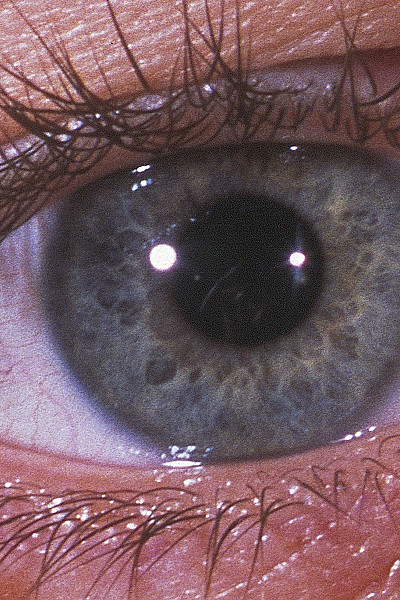The image is an extreme close-up photograph of a human eye occupying the entire width of the frame. The eye belongs to a person with white skin, visible at the top and bottom of the image, where fine, black eyelashes are curving outward. The upper eyelid appears slightly wrinkly with a peach hue, while the lower eyelid matches the skin tone but is less prominent. The eye itself is a light blue color with hints of green, exhibiting a complex, textured pattern radiating outward from the dark black pupil, interspersed with both dark and lighter patches, resembling a marble. Reflections of two bright lights can be seen in the pupil: a smaller reflection on the right and a larger one on the left, indicating a glossed, damp surface. The sclera, or white part of the eye, is detailed with numerous thin red blood vessels, particularly on the left side. The overall clarity and professional quality of the photograph suggest it could have been taken for a medical purpose, possibly in an eye hospital.